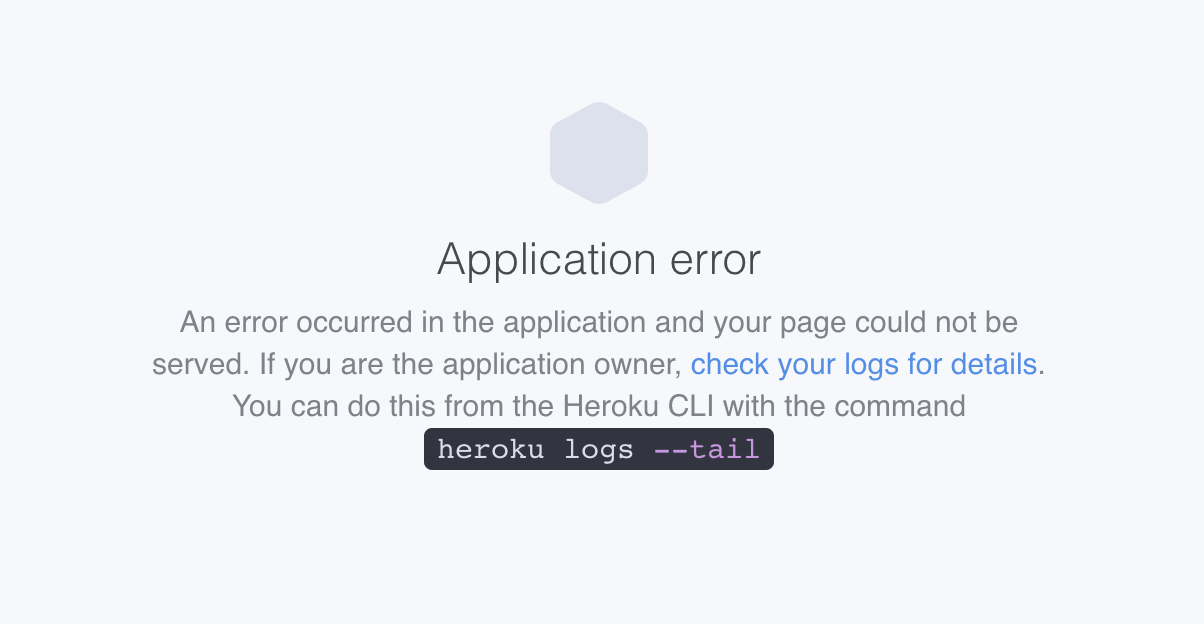This image showcases an application error page, spanning the entire screen in a light gray background. At the top, there is a small gray icon resembling the outline of a rounded box, though the actual box is not visible. Beneath this icon, a bold header displays the words "Application Error." Following this, a detailed message explains the situation: "An error occurred in the application and your page could not be served. If you are the application owner, check your logs for details." Notably, the phrase "check your logs for details" is highlighted in blue, indicating that it is clickable for further information. Additionally, a black box at the end of the paragraph provides a specific command for Heroku users: `heroku logs --tail`. This text is formatted for user interaction, allowing users to copy the command easily. The name "Heroku" is emphasized by its unique spelling, "H-E-R-O-K-U."